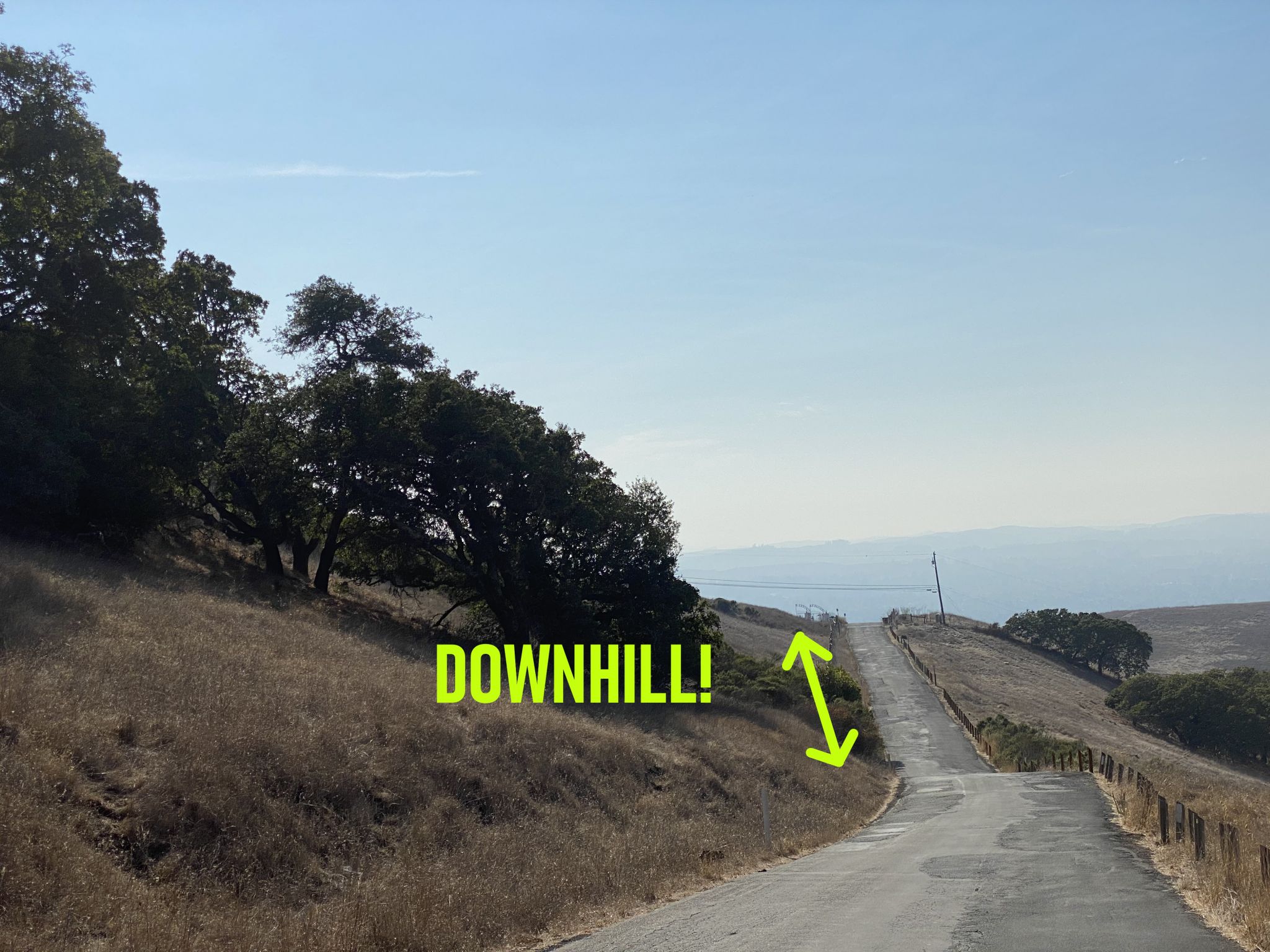The photograph captures a rural, winding road stretching from the bottom right to the center of the image and ascending towards a distant hill. On both sides of the road, there are dry, tan-colored grassy hills adorned with dark green, short, and stubby trees, reflecting a desert-like environment. The smooth, gray pavement has darker indentations in some areas. A tiny, wooden brown fence lines the right side of the road, parallel to the grassy slope. In bright green lettering, the word "DOWNHILL!" is prominently displayed on the road, accompanied by an arrow pointing up and down, indicating the gradient change. The sky is a vivid blue with only a few scattered clouds, and in the background, light blue hills and mountains can be seen, blending into the bright sky.